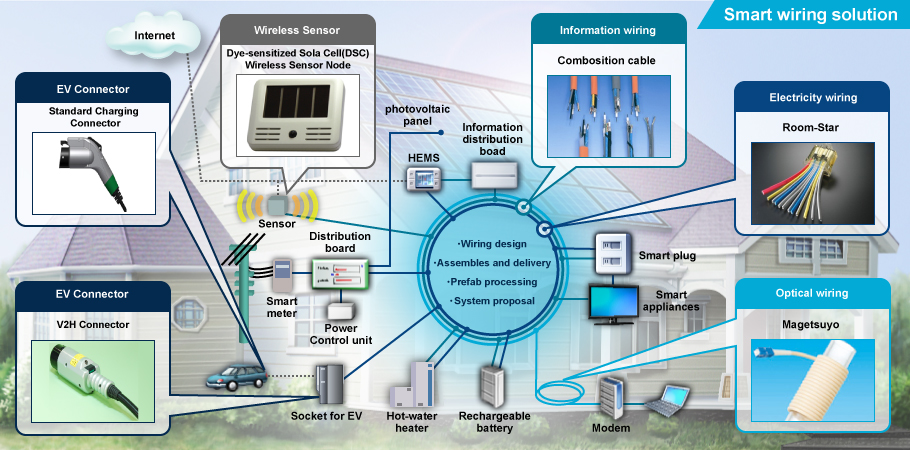This detailed diagram illustrates a comprehensive smart wiring solution for a home, centering around a blue circle that highlights the main processes: wiring design, assembly and delivery, prefab processing, and system proposal. Surrounding the blue circle are various icons representing devices integral to a modern smart home, including an information distribution board, photovoltaic panels, HEMS (Home Energy Management System) devices, distribution boards, sensors, a smart meter, an electric car, an EV charging socket, a hot water heater, a rechargeable battery, a smart plug connected to a smart TV, and a modem with a laptop. 

Encircling these device icons are larger bubbles that denote different types of wiring, such as an EV connector, V2H (Vehicle to Home) connector, standard charging connector, wireless sensor, dye-sensitized solar cell wireless sensor nodes, information wiring composition cable, electricity wiring room star, and optical wiring. All these elements form an interconnected network, indicating the various types of cords and their connections within a smart home setup, effectively tying together energy management, device monitoring, and efficient power distribution through sophisticated wiring solutions.